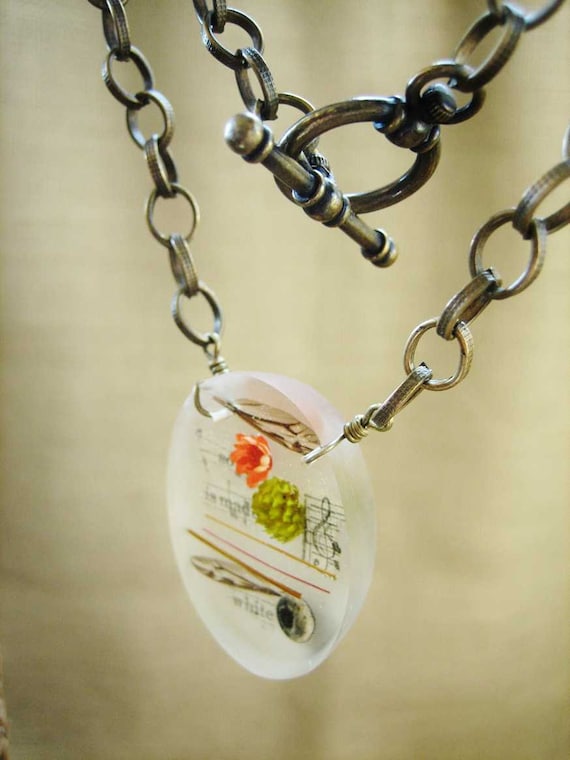This close-up photograph features a unique piece of handmade jewelry, potentially a necklace but not definitively so, suspended in the frame. The chain comprises small, perfectly linked circles forming a V-shape, extending outwards to the left and right edges of the image before converging back towards a clasp. The clasp is a large circle with a T-bar mechanism, suggesting it serves a more functional role if worn around the neck.

At the focal point, a delicate pendant hangs near the bottom center. The pendant is a white circle, angled slightly such that its complete design isn't fully visible. However, within this circular piece are intricate prints, including a recognizable music note and some hard-to-read text that appears to include the word "white." Embedded within the pendant are tiny, meticulously crafted succulents, no larger than the tip of an eraser. One succulent is green, and another is a reddish-peach hue. Additionally, there are small, indeterminate objects and three lines in yellow, red, and brown, running across the pendant, adding further complexity and color to the intricate design.